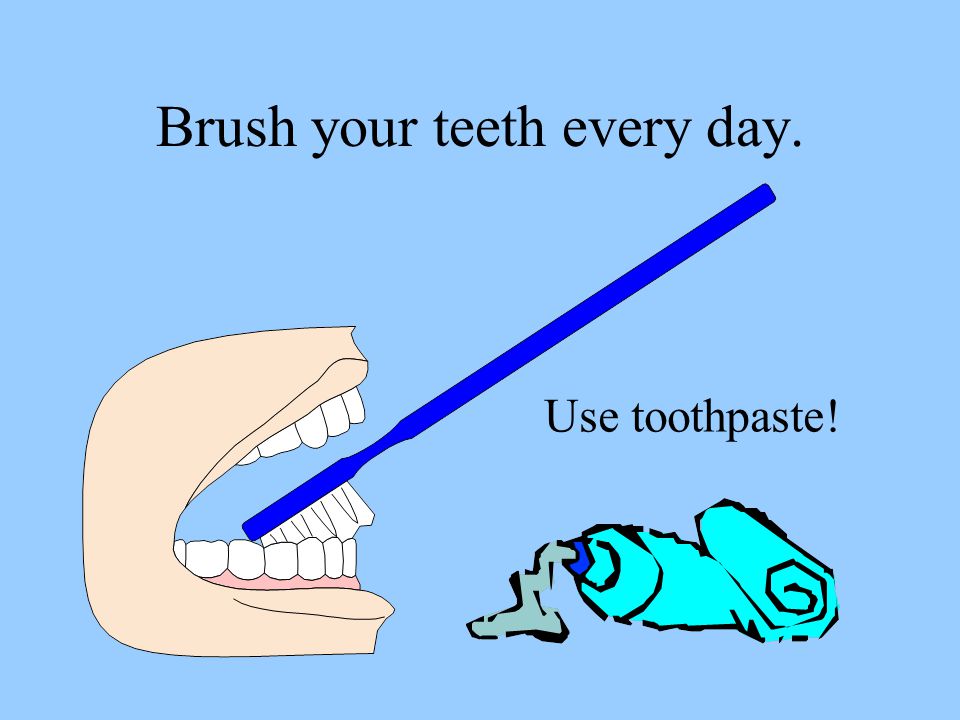The poster features a light blue background with the prominent black text "Brush your teeth every day" centered at the top. Below this, in smaller text, it reads "Use toothpaste!" Positioned towards the left side of the poster is a detailed illustration of an open mouth with visible white teeth—five on the top and seven on the bottom. The gum line is prominently pink but is only visible for the bottom teeth. Leaning diagonally downward towards the bottom teeth is a bright blue toothbrush, with white bristles brushing the back side of the teeth.

To the right of the mouth, there is a turquoise tube of toothpaste, rolled up into a coil, dispensing a squirt of toothpaste. The toothpaste color appears to be a dark, dull green with hints of mint green. The overall design emphasizes the importance of daily dental hygiene using visual and textual elements. This type of poster is likely found in a dentist's or doctor's office to encourage proper dental care practices.